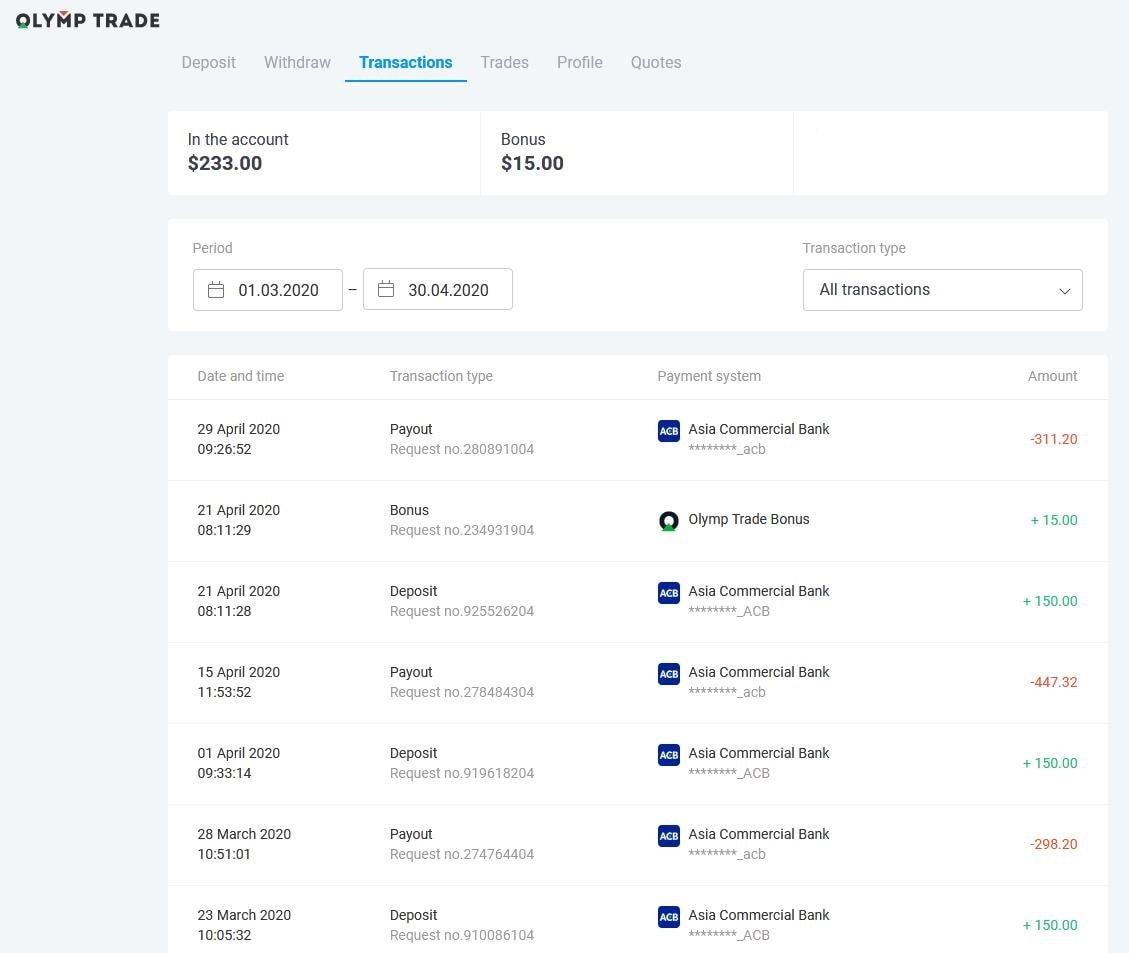A detailed account summary is displayed, showcasing various financial transactions. The summary includes blue-highlighted deposit withdrawal transactions and trades with profiles and quotes. The account balance is noted as $233 with a $15 bonus. The period covered ranges from January 1, 2020, to April 3, 2020.

### Sample Detailed Transaction Breakdown:

- **Transaction Type:** All Transactions
- **Details Displayed:** Date and Time, Transaction Type, Payment System, Payment Amount

#### Transaction Entry (April 29, 2029):
- **Transaction Type:** Payout
- **Request Number:** Referenced by 'NL' followed by a unique number
- **Payment System:** Marked by a blue square icon with the initials 'ACS'
  - **Bank:** Asia Commercial Bank (with additional notation ACB)
- **Amount:** -$311.20 (in red) indicating a deduction

#### Transaction Entry (April 21, 2028):
- **Time:** 11:29
- **Transaction Type:** Bonus
- **Request Number:** OLYMP trade bonus (followed by a unique number)
- **Amount:** +$15.00 (in blue) indicating an addition

The details meticulously outline each transaction with respective amounts, providing a comprehensive understanding of the financial activities within the specified period.